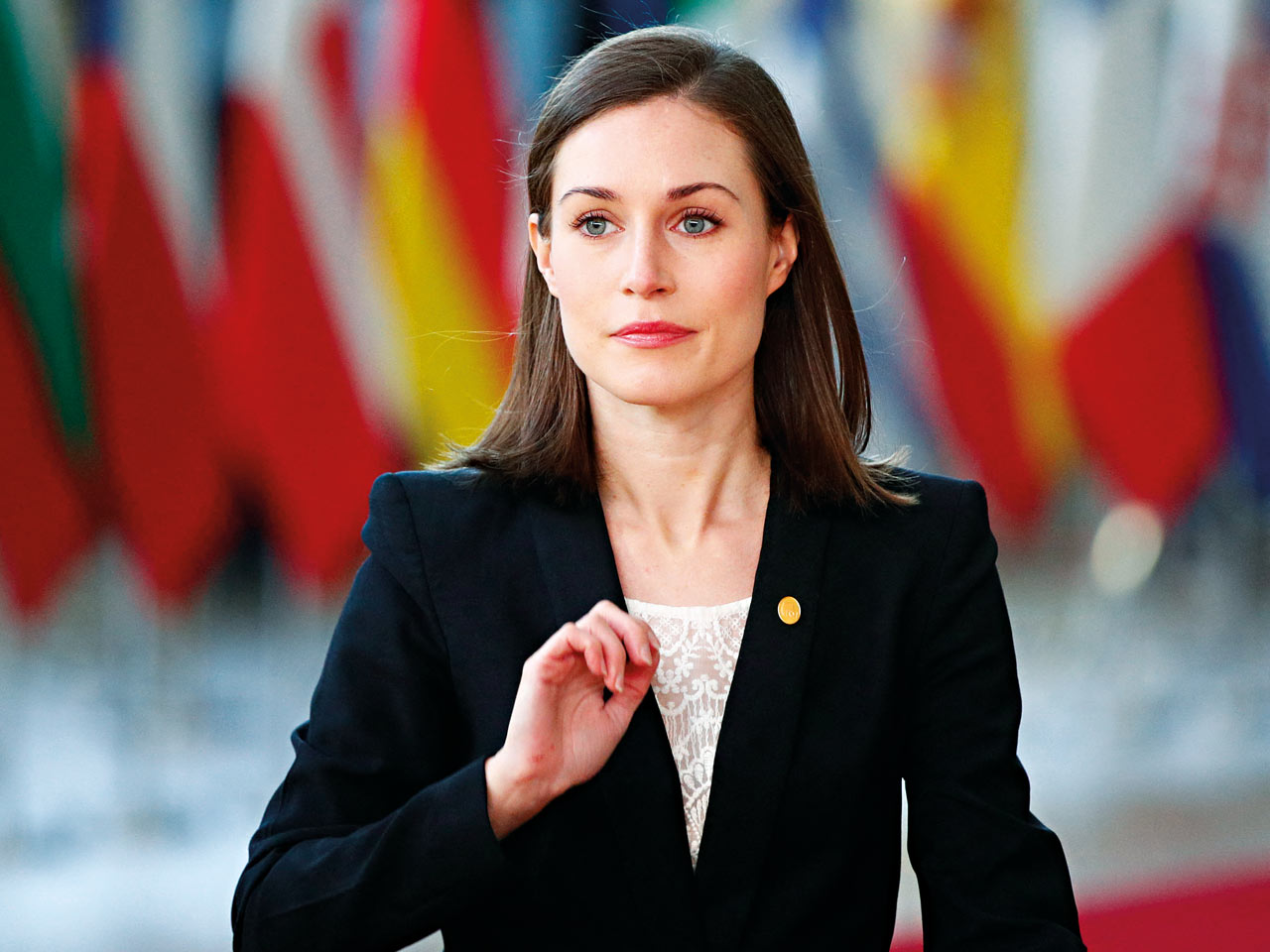The image features a composed woman, who appears to be the former Finnish Prime Minister Sanna Marin, standing waist-up against a backdrop of blurred international flags in various colors such as red, yellow, blue, green, and white. She is wearing a dark blue suit jacket over a white, slightly sheer blouse with a floral or plant print. Her suit jacket sports a gold circular lapel pin on the left side. Her shoulder-length brown hair is parted to the left, and she has blue eyes and light red lipstick, with minimal makeup overall. She is raising her right hand, which is not fully open nor clenched. Her refined features, absence of earrings, and poised demeanor suggest she is either about to speak or looking for someone in the room. The overall clarity of her attire and appearance contrasts with the intentionally blurred flags, emphasizing her central role in the setting.